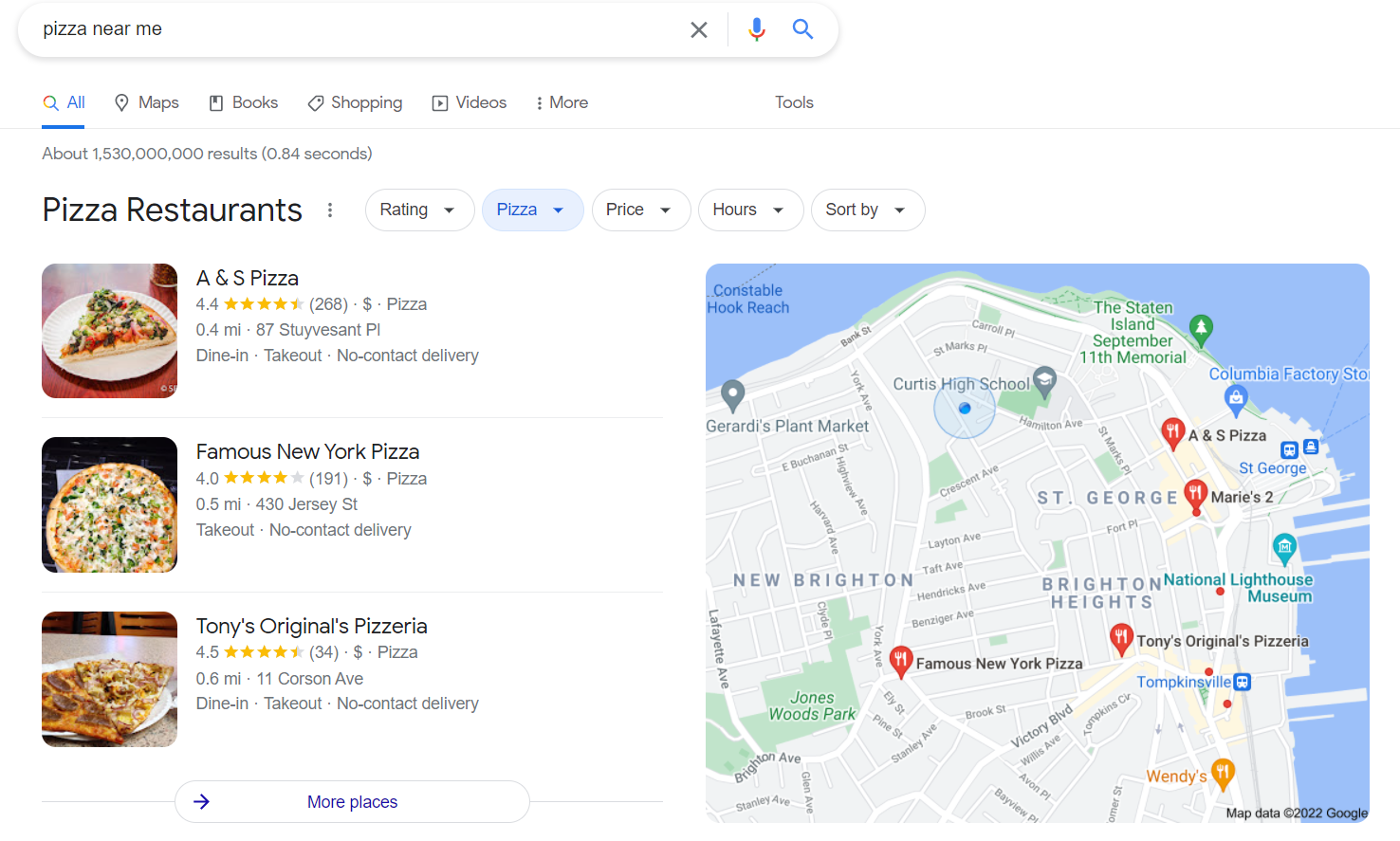In this image, we see a web page displaying search results for "pizza near me." At the very top, there is a search bar with the query "pizza near me" displayed in black text. To the right of the search bar are an 'X,' a microphone icon, and a magnifying glass icon representing another search bar.

Below the search bar, the "All" category is highlighted in blue, indicating the active section. To the right are other category options: "Maps," "Books," "Shopping," "Videos," "More," and "Tools," aligned towards the right. 

Directly below this navigation bar, the search results note approximately 1,530,000,000 results found in 0.84 seconds. The header "Pizza restaurants" is presented in bold black text. Three specific pizza restaurant options are listed: A&S Pizza (rated 4.4 out of 5 stars), Famous New York Pizza (rated 4.0 out of 5 stars), and Tony's Original Pizza (rated 4.5 out of 5 stars). Each listing includes a thumbnail image of pizza, the respective restaurant's address, and the distance from the user's current location. At the bottom of the list is a blue arrow linking to "More places."

On the right-hand side of the page, there is a map featuring the searched area. The map displays blue water areas on the top and right-hand side and light gray land areas with numerous street names. The locations of the three pizza restaurants are marked with red icons, visually indicating their positions on the map.